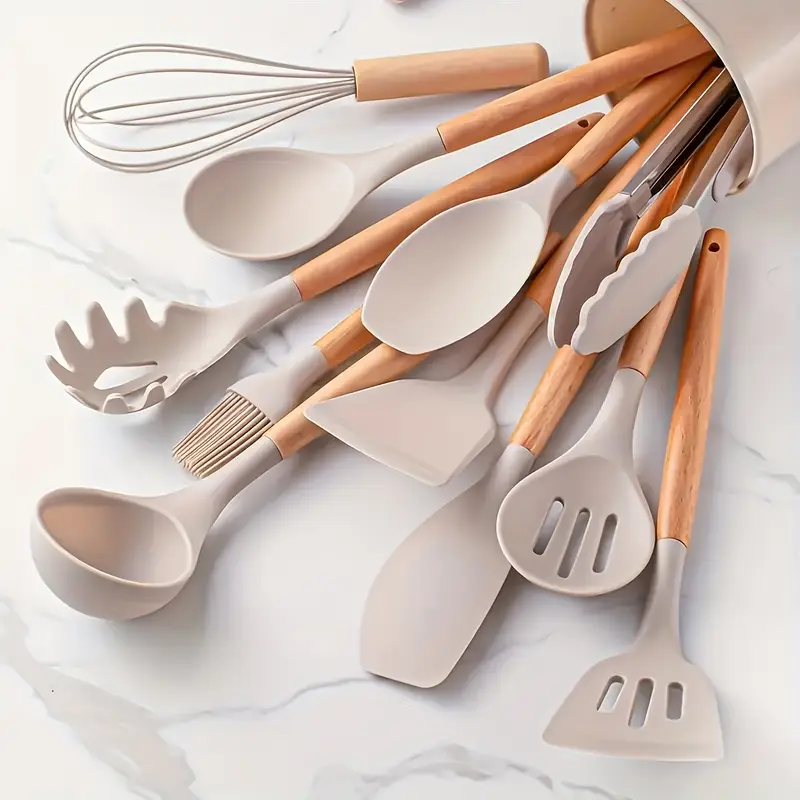The image captures a close-up view of a kitchen counter, detailed with a marble-like white surface accentuated by subtle gray veins. On this counter, a variety of beige cooking utensils with wooden handles are scattered, having spilled out from a white cup tipped over on its side at the top right of the frame. The utensils, arranged at an angle with the handles pointing approximately to the top right, include a diverse assortment: a whisk, a soup ladle, a silicone brush for braising ribs, several spatulas, a large spoon, tongs, and a mixing tool for batter. Some of the utensils, such as a whisk and tongs, remain partially inside the cup, while the rest splay across the countertop, showcasing the comprehensive array of tools essential for a well-equipped kitchen.